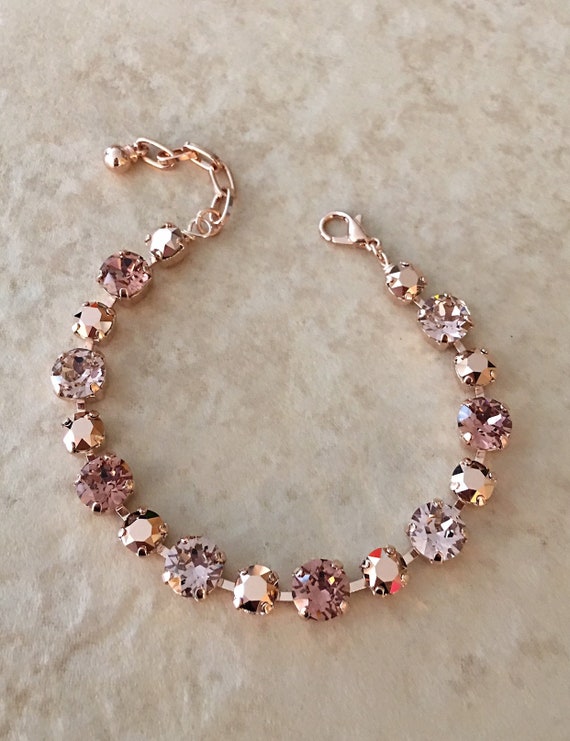The image features a rose gold bracelet adorned with an array of multicolored faux diamonds, including shades of pink, silver, and clear. Each gemstone is meticulously inlaid along the bracelet's chain, which secures around the wrist with a classic clip closure. The bracelet's metalwork has a pink-gold hue, possibly indicating a rose gold overlay on sterling silver. The photo's backdrop is an intriguing beige or tan surface that resembles a marbled or quartz countertop, with a unique, grainy texture akin to halved soap, providing a striking contrast to the bracelet's sparkle. This piece, likely made from costume materials such as cubic zirconia, offers an affordable touch of elegance for those seeking a lower-end luxury accessory.